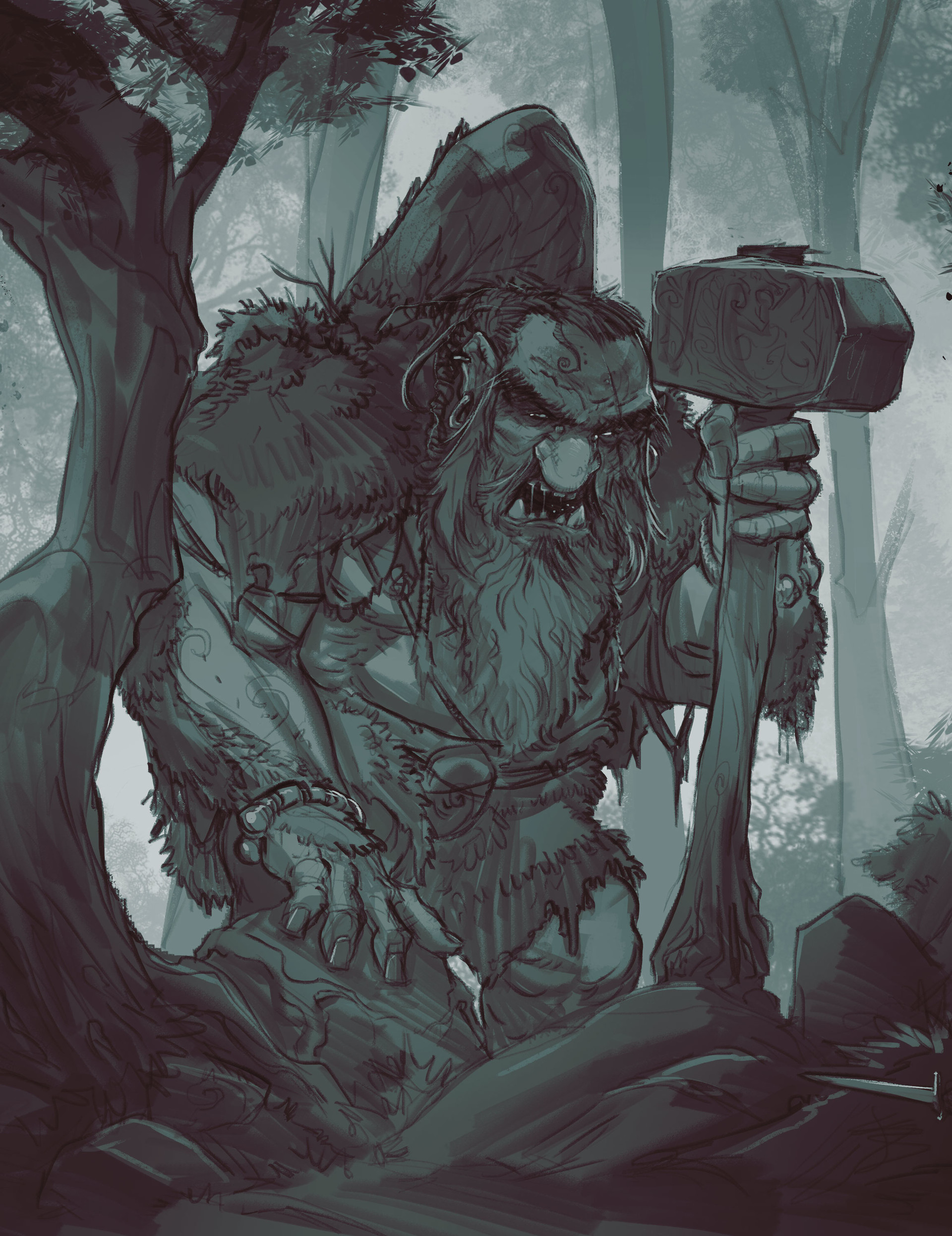This digital drawing presents a formidable ogre-like creature in a monochromatic forest scene. The artwork predominantly employs various shades of gray, with nuances that carry subtle hints of green and blue, creating a somber and somewhat eerie atmosphere. The ogre, with a thick build and a heavy beard, is depicted in mid-stance alongside towering trees and scattered boulders. Its angered expression is emphasized by a pronounced scowl, and a noticeable hunch or protrusion marks its back, adding to its menacing presence.

In its left hand, the ogre brandishes an imposing sledgehammer with an anvil-like head, while its right hand rests on a nearby boulder, highlighting its immense strength. A bracelet adorns its right wrist, suggesting some semblance of adornment or perhaps a hint of its origin. The creature’s attire and overall aesthetic evoke themes of Norse mythology, giving it a mythic and timeless quality.

Despite a lack of a visible artist signature, the effort put into detailing the ogre and its surroundings signals a work of concept art, possibly intended for a game or a broader artistic project. The forest, with its tall trees and shadowy tones, wraps around the ogre, enhancing the feeling of a dark, mythical setting.